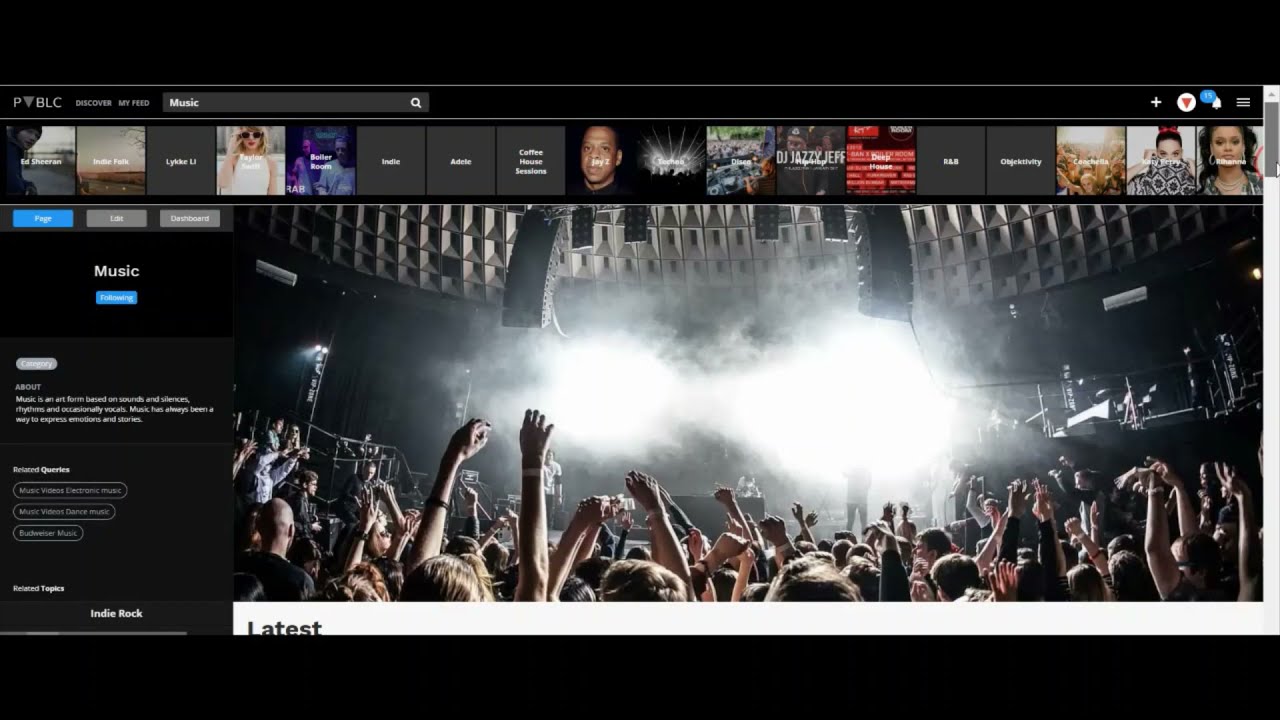A screenshot of a desktop computer display captures an online page with a black background. Dominating the center of the screen is a large photo of an electrifying concert. The image showcases a sea of concert-goers from behind, with countless hands raised high into the air, contributing to the exhilarated atmosphere. The stage, enveloped in a haze of smoke effects and vibrant light displays, has a predominantly grey backdrop. 

Above the main concert image is a horizontal strip featuring several small images, each depicting different performers, likely singers. On the left side of the concert photo, the word "MUSIC" is prominently displayed in white text. Directly below this word is a distinctive blue button. Further down, smaller white text provides additional information, though it is not legible from the screenshot.